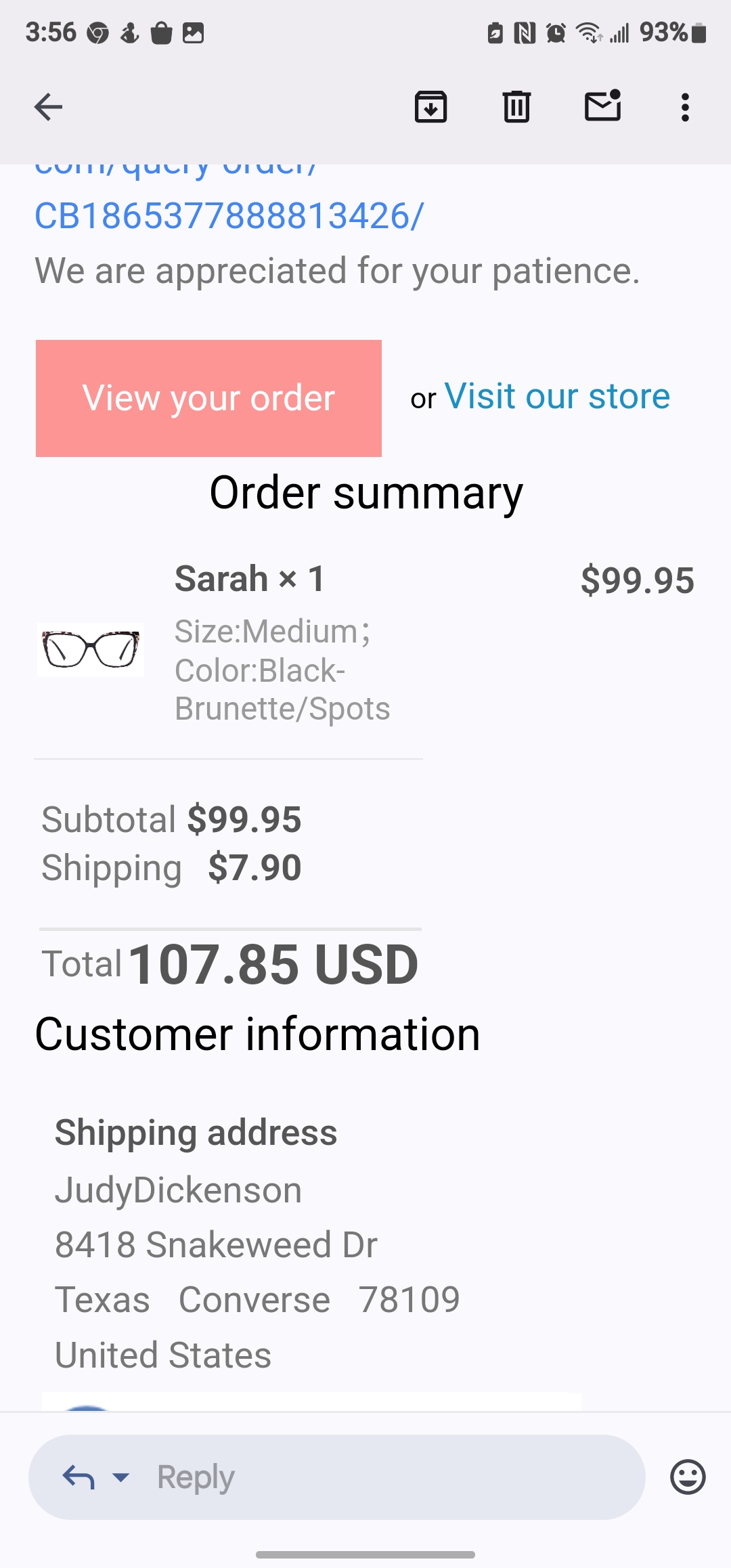The image depicts a smartphone screen displaying an order summary from an eyeglasses website. At the top of the screen, the time is shown as 3:56, accompanied by a series of small icons including a Google icon, a ringer icon, and more, with a battery icon indicating 93% charge, a Wi-Fi icon, a signal bar icon, and other less recognizable icons all within a light gray bar. 

Within this bar, on the left side, there is a back arrow, and on the right side, there are icons for folder options, deletion (trash can), email or sending (envelope), and a three-dot menu. Beneath this bar, part of a URL appears, showing ".com/query" and an alphanumeric string. 

The main body text reads somewhat awkwardly, likely due to translation from another language: "We are appreciated for your patience." Below this, there is a coral pink-red rectangle with white text saying "View your order," and next to it, a clickable blue link that says "visit our store."

The order summary details reveal that the item ordered is "Sarah" eyeglasses, quantity one, with a small thumbnail image of the glasses. The specifications include size Medium and color described as "Black-Brunette/Spot," suggesting a tortoise shell frame, for $99.95. The subtotal is listed as $99.95 with a $7.90 shipping cost, bringing the total to $107.85 USD.

Under the "Customer Information" section, the shipping address, bolded, is Judy Dickinson, 8418 Snakeweed Drive, Texas, Converse 78109, United States. Note that the state and city are incorrectly placed.

At the bottom of the screen, there is a chat function with a reply box and an emoji icon, indicating an option to interact with customer service. The rest of the page is cropped off.